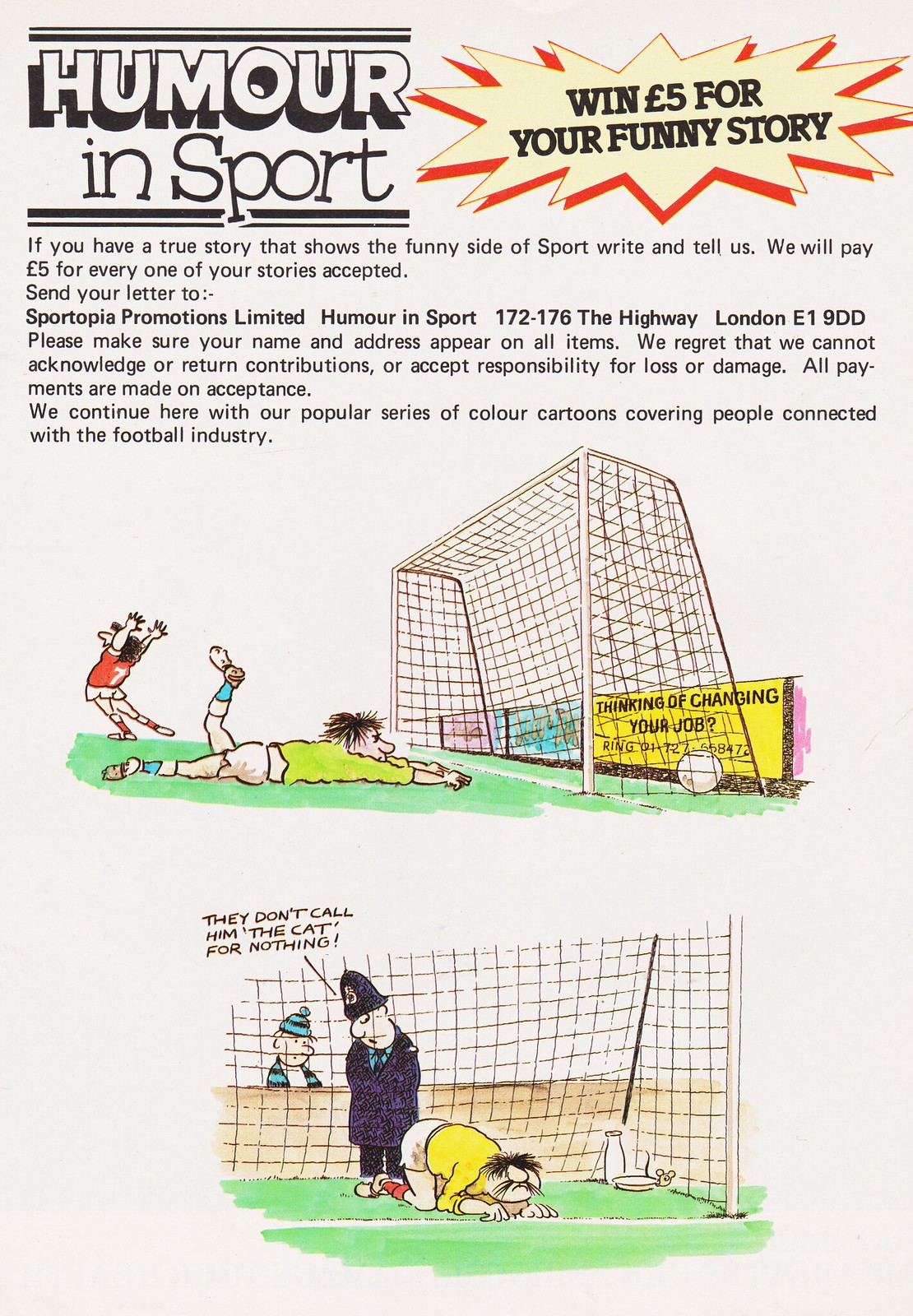The page, likely from a sports magazine or program, features a light gray background with a hand-drawn headline in the upper left corner that reads "Humor in Sport" in large block white letters with a shadow behind them. To the right of the headline, there is a yellow star with red shadowing, accompanied by the text, "Win five pounds for your funny story." Below this headline, a detailed paragraph invites readers to submit their true, humorous sports stories, promising a payment of five pounds for each accepted entry. Contributions are to be sent to Sportive Promotions Limited at 172-176 The Highway, London EY9DD, with a note that the sender’s name and address should be included on all submissions. The text clarifies that they cannot acknowledge or return contributions nor accept responsibility for loss or damage, and that payments are made upon acceptance.

Below this, the page continues with a popular series of color cartoons related to the football industry. The first cartoon depicts a humorous scene where a soccer goalie, dressed in a green shirt, is laying on the ground with one foot up in the air, having missed a save. In the background, a red-jerseyed player, number seven, is seen celebrating with arms raised, while his stomach notably sticks out to the left, emphasizing the comic mishap. The second cartoon shows a police officer inside the goal, with a person in a yellow shirt down on hands and knees in front of him. Above the officer, text reads, "They don't call him 'the cat' for nothing," adding to the humor as a bottle of milk and a saucer are seen in the back corner of the goal, playfully suggesting the goalie's cat-like crouch. The detailed, whimsical captions and illustrations highlight the lighter side of sports, inviting readers to engage with their own comical experiences.